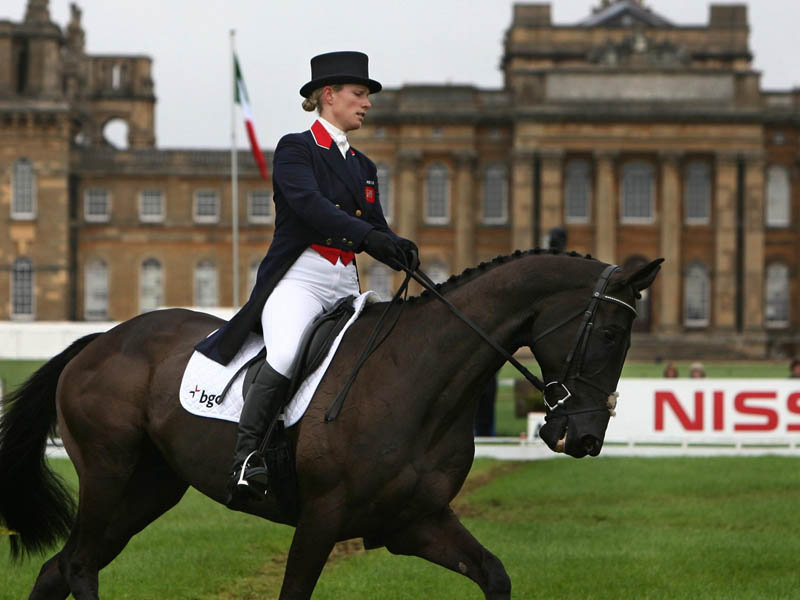This image depicts the professional equestrian Zara Tindall as she participates in a formal equestrian event. Zara is elegantly dressed in black riding boots that reach her knees, white pants, black gloves, and a black blazer-style coat with tails and a red lapel that transitions to blue or black nearer to her chest. Completing her outfit, she wears a white handkerchief tied into a bow at her neck and a black top hat. Her hair is neatly styled in a bun at the back. She rides a strong, young horse with a very dark brown or black coat and a braided mane, equipped with a dark saddle and a white blanket underneath. The background features a grand building reminiscent of a palace, with multiple rows of windows and tall brick columns. The scene is set on a lush green grass field under a mostly gray sky with some patches of white and blue. Additionally, there is a flag on a pole and a white sign displaying "NISS" in red letters, possibly indicating the Nissan logo. The overall atmosphere suggests a prestigious and serene event.